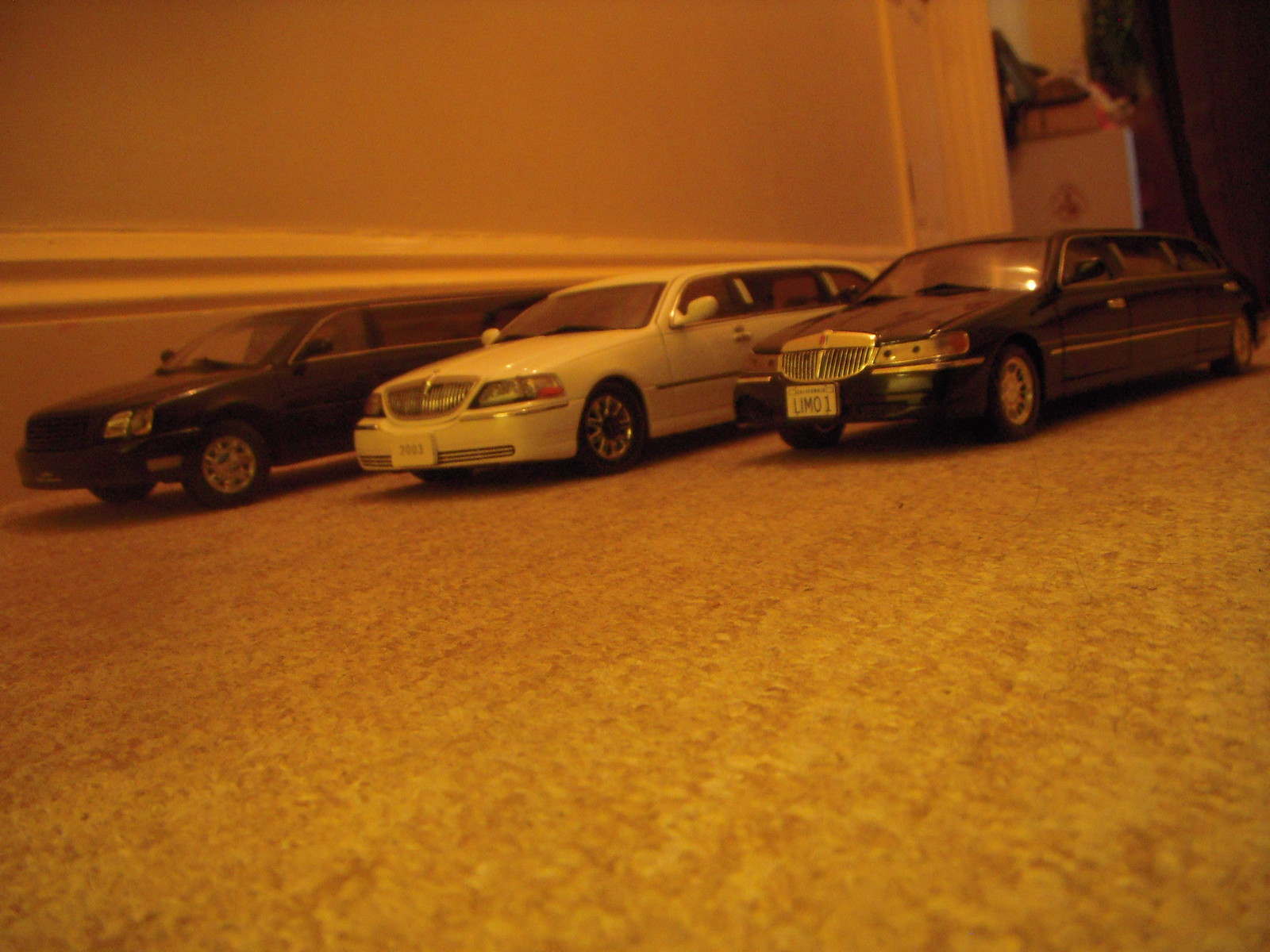This close-up color photo features three toy limousine cars meticulously arranged on a carpeted floor that appears to have an orange or yellow tint due to the lighting. The cars are positioned parallel to a white baseboard against a lightly colored, shadowy wall, suggesting the photo might have been taken in low light conditions, possibly at night. The formation of the cars mimics a staggered race lineup, with two black limousines framing a white one, each sporting distinct front features—a shiny silver grill on two, while the third, nearest to the wall, lacks this detail. Notably, the black limousine to the left displays a legible license plate reading "LIMO 1," while the plate on the black limousine to the right seems to read "3003," and the third plate is indiscernible. The background shows some clutter, including a glimpse of a doorway, possibly boxes, and a dark curtain, adding to the scene's everyday, lived-in feel.